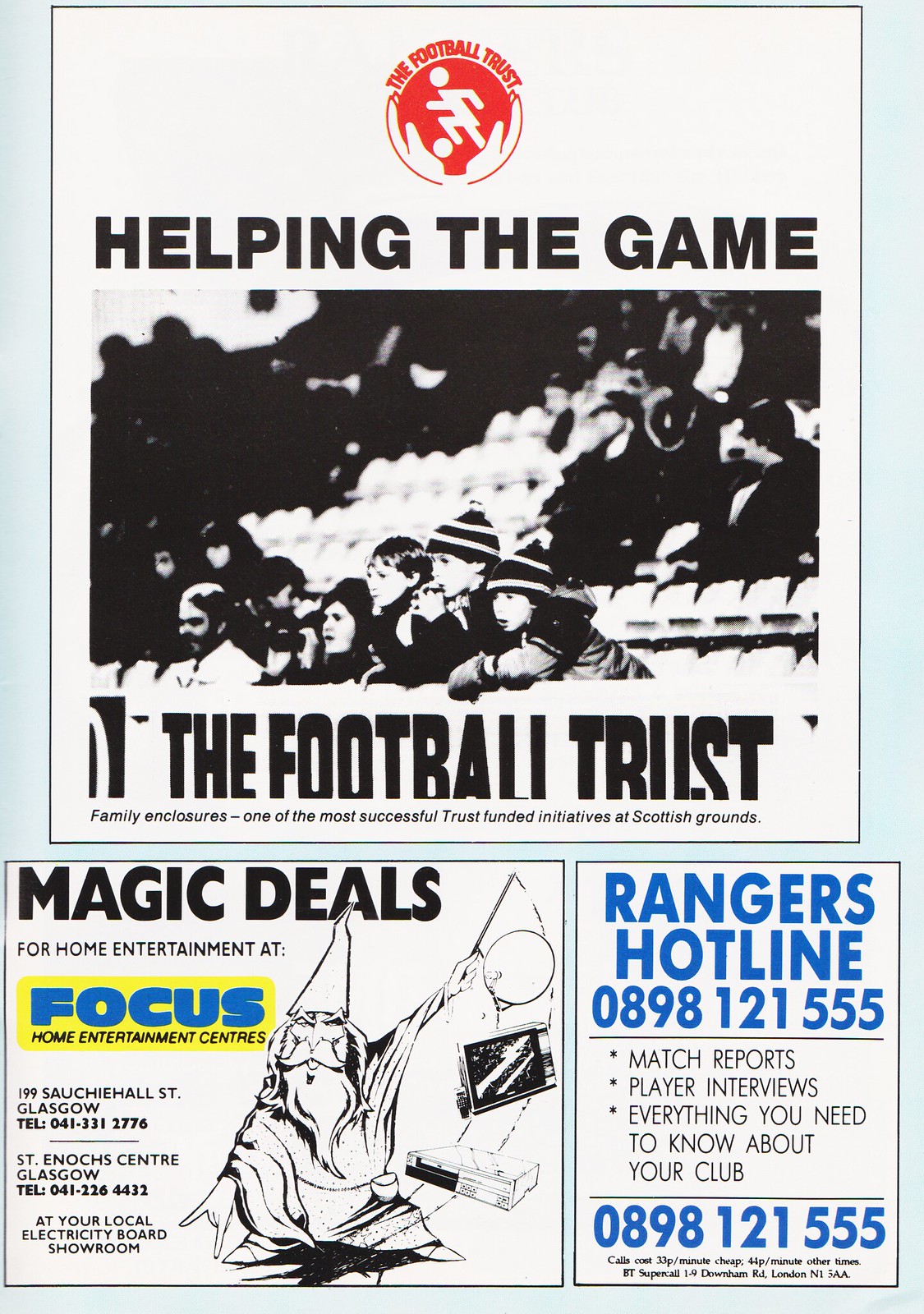The image depicts a vertically aligned rectangular poster, likely extracted from a football magazine titled "The Football Truist." The background is a very light blue, visible mainly at the top corners. Dominating the top section is a large white square featuring the red circular logo of The Football Trust, depicted with two hands holding a circle and a silhouette of a running stick figure. Curving around the circle, the text reads "The Football Trust." Just below this, in black lettering, is the slogan "Helping The Game."

Beneath the logo and slogan, a black and white photograph captures a group of children in stadium stands attentively watching a football game, with additional spectators visible in the background. Directly under the image, the text mentions "Family enclosures, one of the most successful Trust-funded initiatives at Scottish grounds."

The bottom portion of the poster contains two distinct advertisement sections. On the left, a yellow background square advertises "Magic Deals for Home Entertainment at Focus Home Entertainment Centers," highlighted by "Focus" in large blue letters and an image of a wizard. The right-side square, set against the blue text backdrop, promotes the "Rangers Hotline" with the phone number 0898-121-555. It lists services like "Match Reports," "Player Interviews," and "Everything you need to know about your club," reiterating the phone number in blue text at the bottom. This phone number and other details, along with mentions of Glasgow, confirm the content pertains to European football, specifically Scottish football, rather than American football.